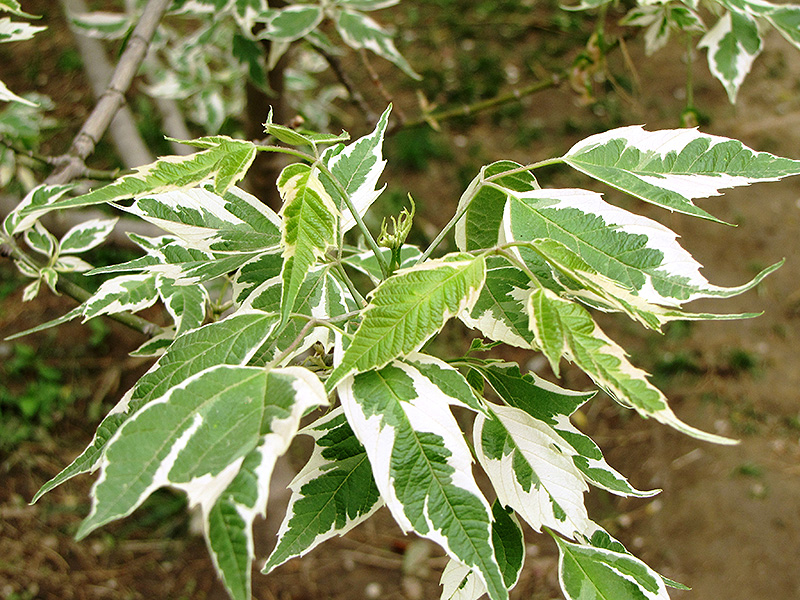This is a close-up nature photograph of variegated leaves from a plant, taken outdoors. The main subject in focus features unique, serrated leaves with a sharp-angled, saw blade-like cut along the edges. These leaves display a variegated pattern, with bright green centers and vibrant white borders; some even have larger patches of white interspersed with green. Attached to thick green stems that appear to sprout from a tree with a notably thick branch in the upper left corner, the leaves extend outward. The background is artistically blurred, showcasing a brown ground interspersed with green grass, fallen leaves, and gray branches, enhancing the focus on the striking foliage in the foreground.